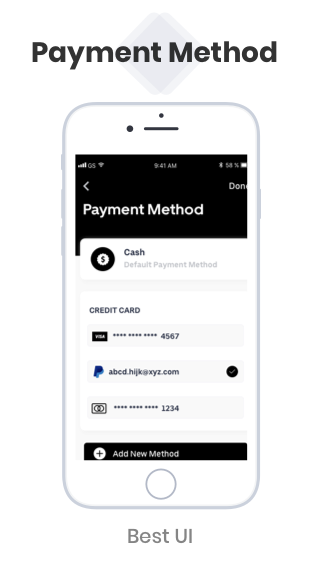An iPhone screen displays a mobile application interface for managing payment methods. At the top of the screen, "Payment Method" is prominently labeled. Below this, "Cash" is listed as the default payment method, represented by a black circle icon featuring a white money symbol inside. The app also offers the option to add other payment methods including credit cards and PayPal accounts. An example PayPal indication appears as "abcd.hijk.xyz.com," serving as a placeholder email address. Credit card entries are indicated by a series of asterisks followed by the last four digits, "4567."

Further down, a money icon suggests the capability to add a debit card, also denoted with asterisks and ending with the digits "1234." At the bottom of the screen, the option "Add New Method" is available, displayed in white text against a black background.

The phone status bar shows it is 9:41 AM, with full Wi-Fi signal, full phone service, 54% battery remaining, and Bluetooth enabled. The bottom of the screen displays a caption "Best UI," indicative of a user interface design commendation.